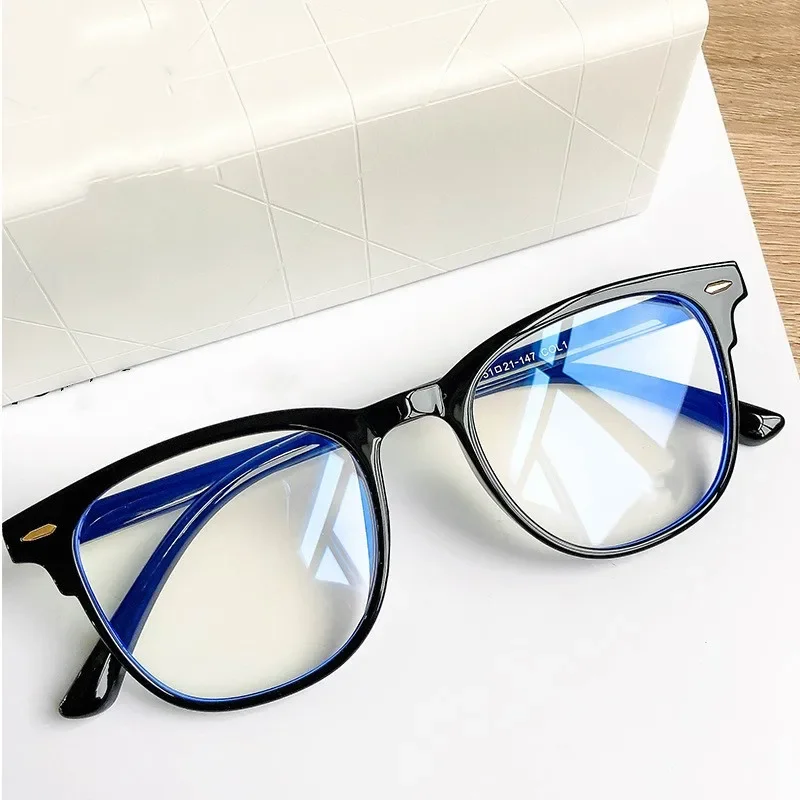This detailed photograph features a stylish pair of black eyeglasses with small, gold horizontal accents on the outer edges of the frames. The glasses, highly polished and reflective, are carefully folded and placed diagonally, extending from the bottom left towards the upper right of the image. They rest on a stark white surface, which could be a piece of paper, against a backdrop that includes a rounded, rectangular white object with etched straight lines at various angles. The surface itself sits on a light walnut-colored wooden table or floor. Intriguingly, the reflection in the lenses reveals a window and partially obscured alphanumeric details on the inside of the glasses' arm, possibly reading "51021-147 COL1". The precise arrangement and gleaming surface of the glasses, along with the soft light capturing intricate details, create an elegant and sophisticated composition.